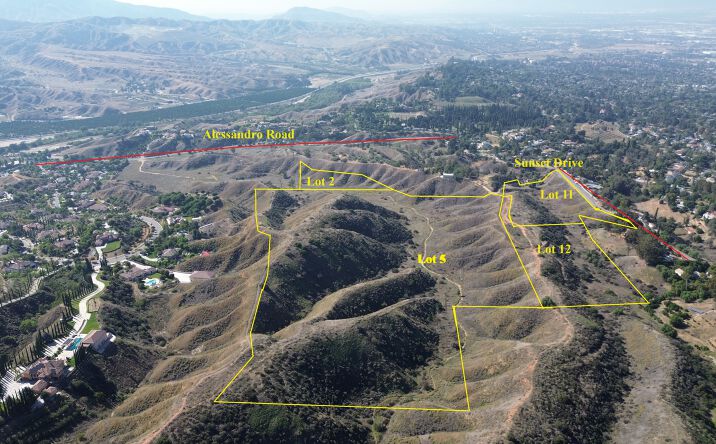This aerial image captures a picturesque expanse of gently rolling hilltops, resembling a low mountain terrain. Nestled within this natural landscape, homes and buildings are scattered to the left and right, extending toward the horizon. Hand-drawn yellow lines demarcate various property lots, clearly highlighting the area for potential development or sale. Notable road names, such as Alexandro Road and Sunset Drive, are marked in red, guiding viewers through the terrain. The largest designated area, Lot 5, encompasses most of the hilltops, while smaller sections like Lot 2, Lot 12, and Lot 11 are also clearly labeled. This detailed illustration provides a comprehensive overview of the available lots within this serene and expansive environment.